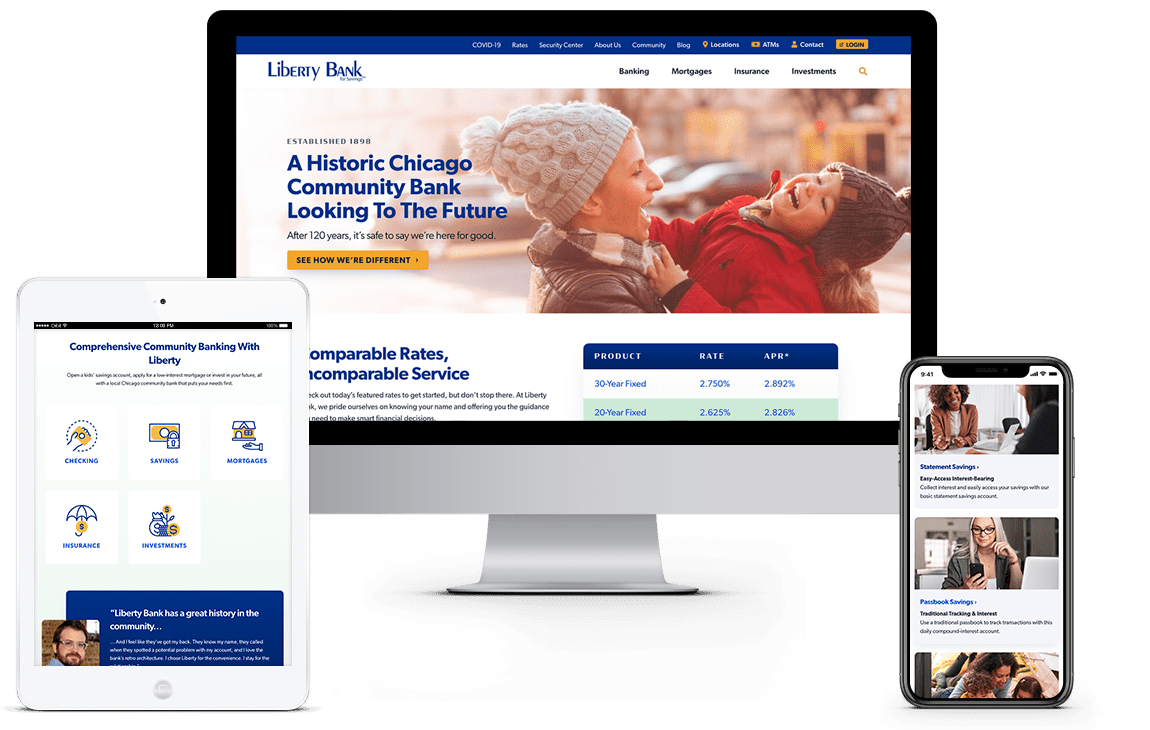This advertisement from Liberty Bank showcases a desktop, an iPad, and an iPhone displaying various promotional attributes of the bank. Positioned in the upper left-hand corner is the Liberty Bank logo, and prominently featured in the center is an image of a mother and daughter dressed in winter attire— the daughter wearing a red jacket and the mother donning a black leather jacket paired with a plaid scarf. The caption, "A historic Chicago community bank looking to the future," highlights the bank's long-standing relationship with its community and forward-thinking approach. 

A yellow call-to-action line reads, "See how we're different," encouraging viewers to click and learn more about the bank's offerings. Below this, somewhat obscured by the image of the iPad, the text mentions competitive rates and services, reinforcing Liberty Bank's customer-focused philosophy. The tagline, "Comprehensive community banking with Liberty," is emphasized, accompanied by various icons symbolizing the bank's diverse range of services.

Towards the bottom of the image, a testimonial from a man extolls the community-centric history of Liberty Bank, underlining its enduring commitment. The iPhone, leaning against the desktop, shows an image of a Black woman engaged in a professional discussion with another woman at a desk, and another visual of a white woman with blonde hair looking at her phone. The advertisement also includes a photo of a mother with her two children, illustrating the personal connection and trust Liberty Bank fosters with its clients.

The contact options available through the advertisement emphasize the bank's accessibility and range of services including banking, mortgages, and more, inviting potential clients to learn how Liberty Bank can support their financial needs.